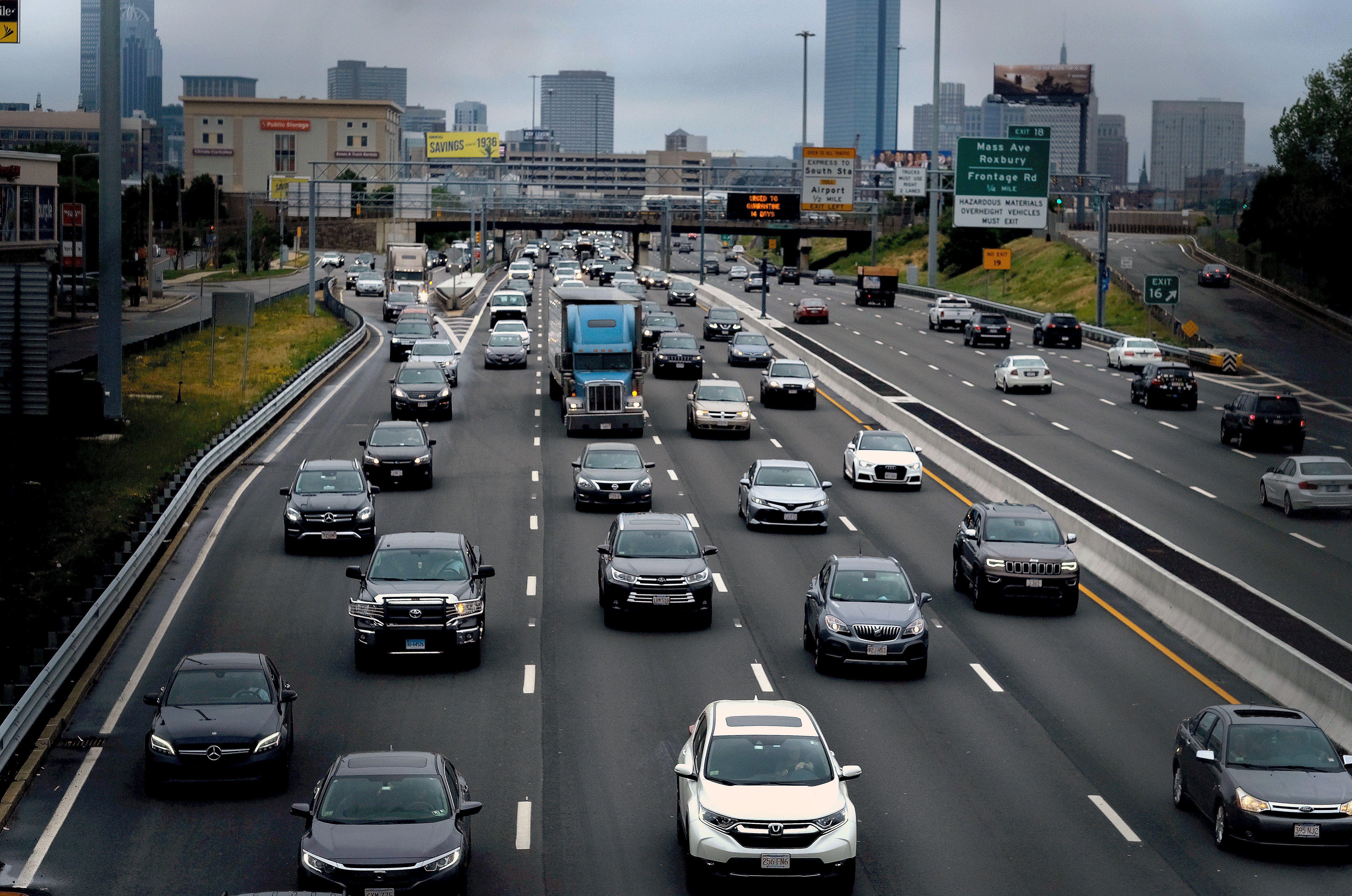This image captures a bustling highway scene in Boston, Massachusetts, likely near Exit 16 and Exit 19, pointing towards Mass Avenue, Roxbury, and Frontage Road. The traffic is particularly heavy on one side of the road, with well over 30 vehicles, primarily in shades of black, gray, and white, with a noticeable bright blue truck and a brown truck in the mix. The highway, adorned with numerous signs, demonstrates the intricate network of roads leading to notable destinations such as South Station and the Airport. The signs also mention hazardous and overheated vehicles, cautioning drivers of potential delays due to road construction. As the roads converge under a bridge, the backdrop reveals the towering skyline of Boston with various tall office buildings and banks. The scene is set on an overcast day, with patches of green and yellow grass lining the roadside, encapsulating the dynamic yet typical traffic flow of a medium to large-sized American city.